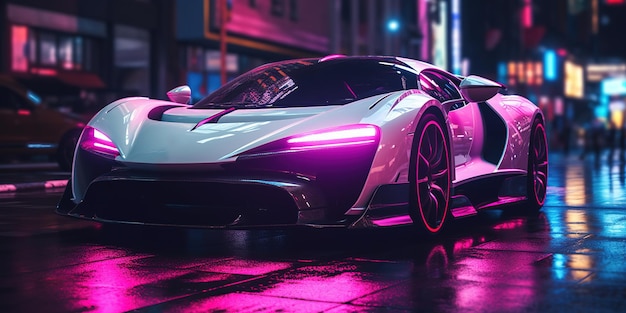The image showcases a highly detailed, digital rendering of a sleek, modern sports car that boasts an eye-catching design under dazzling LED lights. This low-profile car, set against a blurred urban backdrop, exhibits a glossy gray finish with pink and purple hues reflecting off its surface, suggesting the presence of vibrant lighting. The car is adorned with futuristic, upward-opening doors resembling wings, and large, stylish rims complement its sporty appearance. The front grille and windshield, both sharply focused, add to the vehicle’s dynamic look. The wet street beneath reflects the pinkish-purple glow, enhancing the vividness of the scene. In the background, city buildings and indistinct figures are visible under blue LED lights, adding depth without diverting attention from the car.